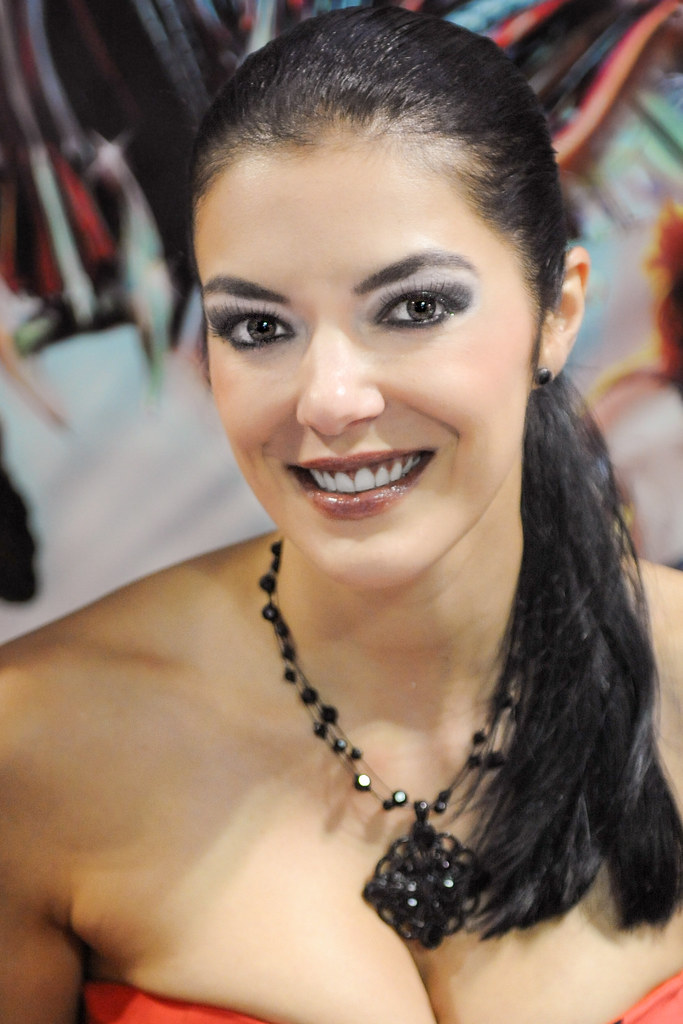This is a tall, rectangular image capturing a young woman from the chest up, taken from a slightly elevated angle. She gazes directly forward with a charming smile, revealing her top teeth. Her long, dark black hair is slicked back into a ponytail that elegantly drapes over her right shoulder. She has green eyes, dark purplish lipstick, and a well-defined facial structure. Her makeup includes black and white eye shadow, complementing her dark blackish-brown eyebrows.

Around her neck, she wears a black beaded necklace featuring a sizable black square pendant hanging off one of its corners. She is dressed in a strapless orange or reddish dress, revealing some cleavage and hinting at a voluptuous figure. Her skin tone is light and fair. The background is a mix of various colors above a predominantly white lower area, possibly including elements resembling flamingos, adding a vibrant and exotic touch to the composition.